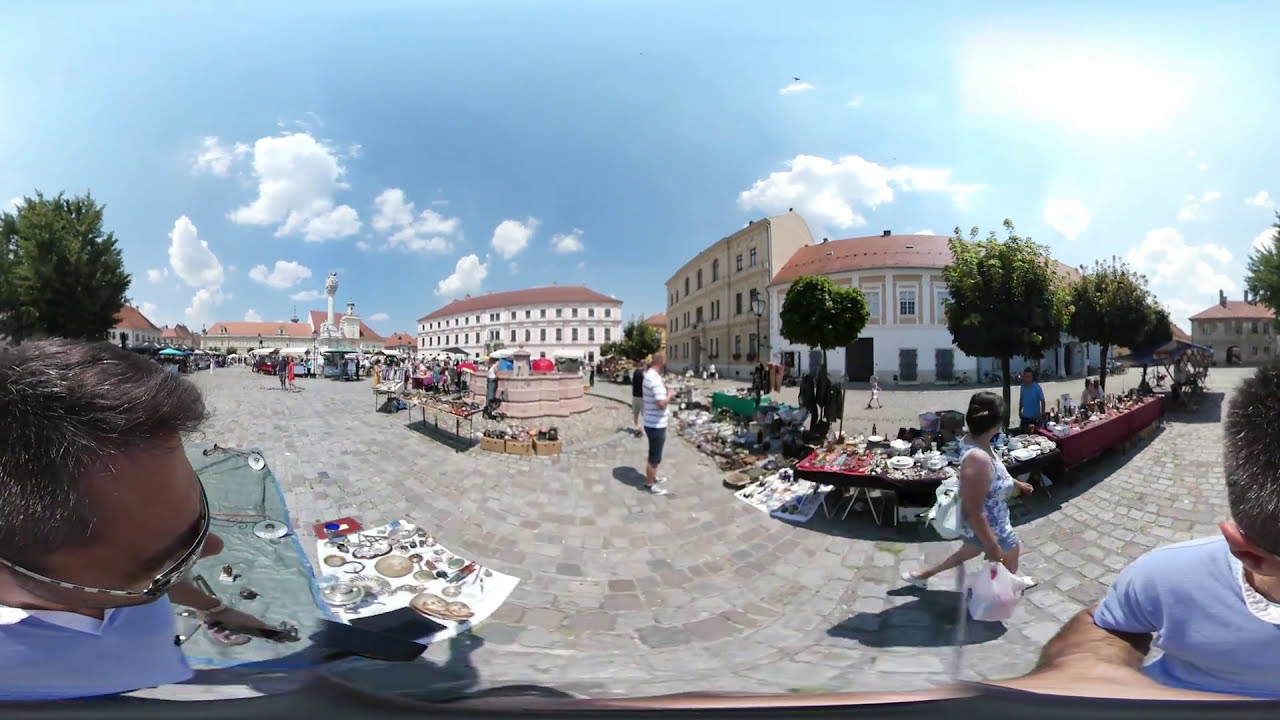This is a panoramic photograph taken outdoors, showcasing a bustling courtyard filled with various vendor stalls. The photo is slightly curved, indicating the use of a panorama or fisheye lens. The photographer, partially visible in the frame, wears a blue shirt and glasses, walking on a path made of grey rectangular bricks. The scene is vibrant with activity; numerous stalls display goods ranging from clothes and shoes to silverware and artisan crafts, resembling a lively street fair or flea market. Several people are milling about— some walking, others browsing or inquiring about the items for sale.

The courtyard is shaded by sporadic trees, and in the background, there are white and beige buildings with reddish-brown rooftops, hinting at European architecture. The sky above is a stunning blue, dotted with white fluffy clouds, and the sun can be seen shining brightly on the right side, casting a warm light over the scene.